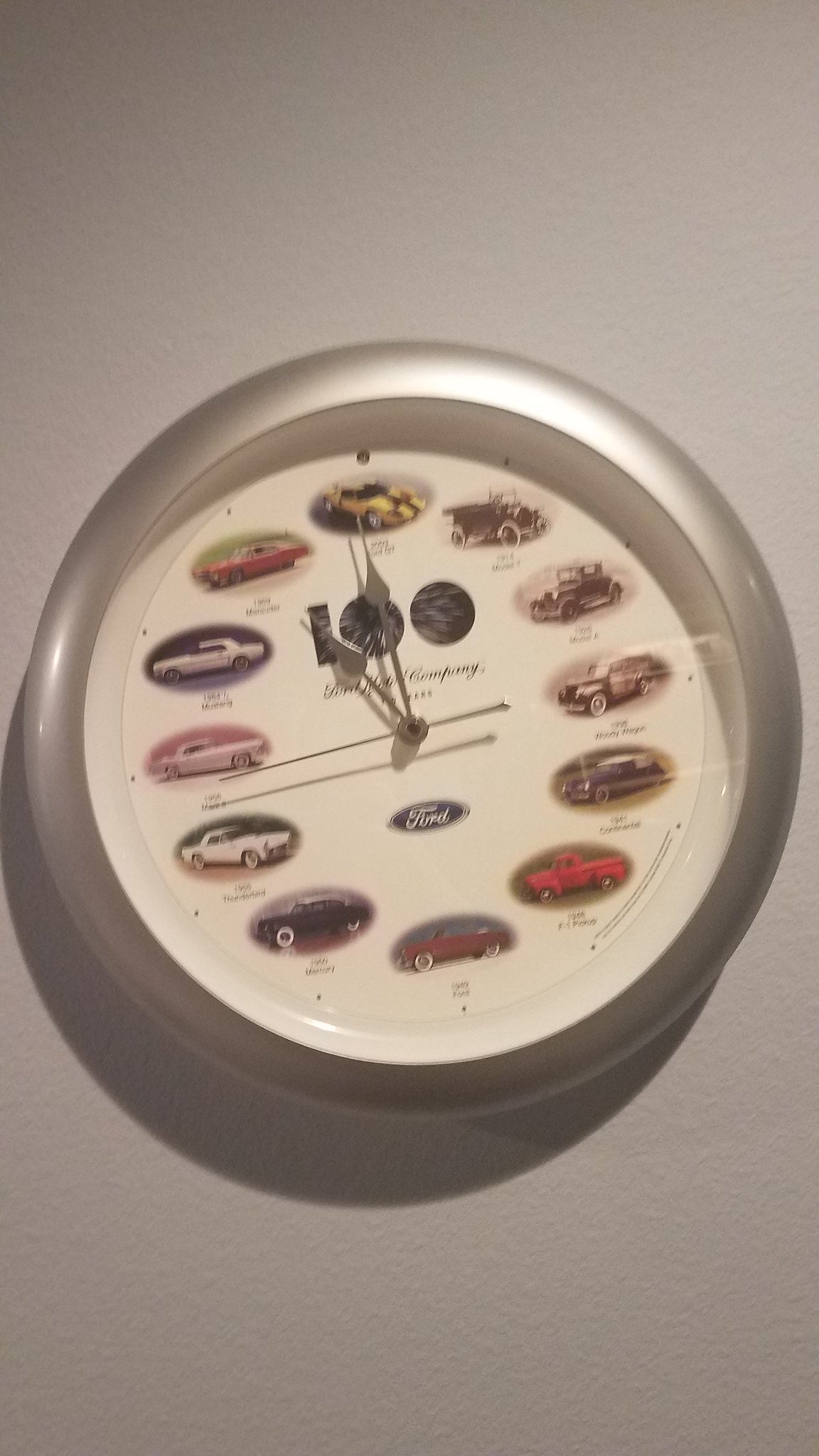The rectangular image, oriented vertically, features a wall clock mounted on a grayish-white wall. The clock is framed in silver, and its face has a cream-colored background. Instead of traditional numbers, the face showcases an oval arrangement of illustrations depicting various antique cars. 

At the 12 o'clock position, there is a yellow sports car with a black stripe. The 1 o'clock position features an antique jalopy-style car. At the 6 o'clock position, a red convertible sports car is depicted. 

The center of the clock houses the silver hands for the minute, hour, and second, along with the text "100 Ford Motor Company." Below the hands, an oval emblem displays the word "Ford" in white text against a black background. A subtle shadow can be seen beneath the clock, adding depth to the image.